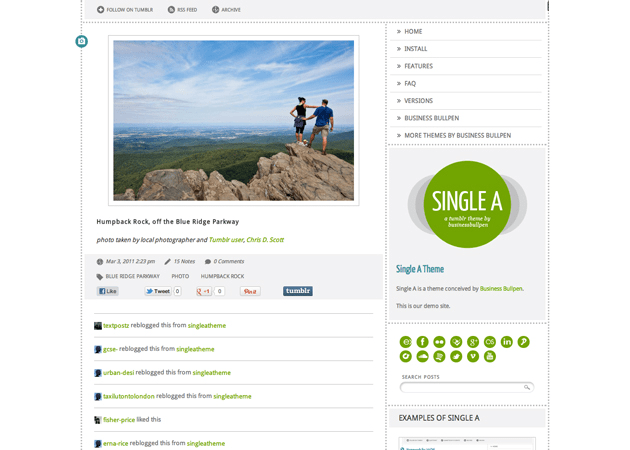The image is a screenshot from a website with a white background and predominantly black text. At the top left corner, there are three buttons labeled "Follow on Tumblr," "RSS Feed," and "Archive." Below these buttons, there's a landscape photograph depicting a couple, a Caucasian man and woman, embracing each other at the summit of a jagged mountainside. The background showcases a sky with clouds, accompanied by green trees and bushes below.

Next to the photograph, there is a vertical menu listing the following sections: "Home," "Install," "Features," "Facts," "Versions," "Business Bullpen," and "More Themes by Business Bullpen." Beneath this menu is a logo consisting of a green circle with a white 'A' inside it and the text "A Tumblr theme by Business Bullpen" in yellow. Below the logo, the text "Single A Theme" is displayed in blue, followed by "Single A Theme conceived by Business Bullpen" in black. This is followed by the statement "This is our demo site."

Further down, there are buttons for social media links including Facebook, Twitter, Indeed, and Google+. To the left of the photograph, there is a caption that reads "Humpback Rock off the Blue Ridge Parkway, photo taken by local photographer and Tumblr user Christy Scott." Additional details include various timestamps, zero comments, and buttons for liking on Facebook, tweeting, and sharing on Tumblr. Below this section, there are about six interactions, such as reblogs or likes by different people.